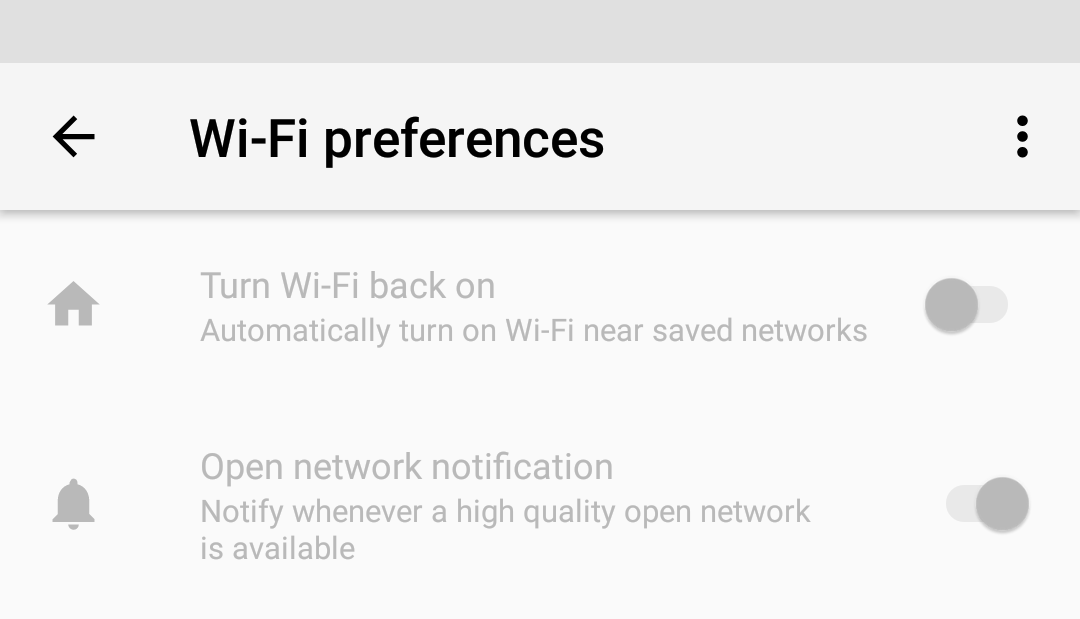The image displays a computer settings screen with a light gray background. At the top in bold black text, it reads "Wi-Fi Preferences." Beneath this heading is an option labeled "Turn Wi-Fi back on automatically," followed by another option titled "Turn on Wi-Fi near saved networks," which is currently toggled off. Below these settings, there is a feature named "Open Network Notification" with a description that says, "Notify whenever a high-quality open network is available." This option is toggled on.